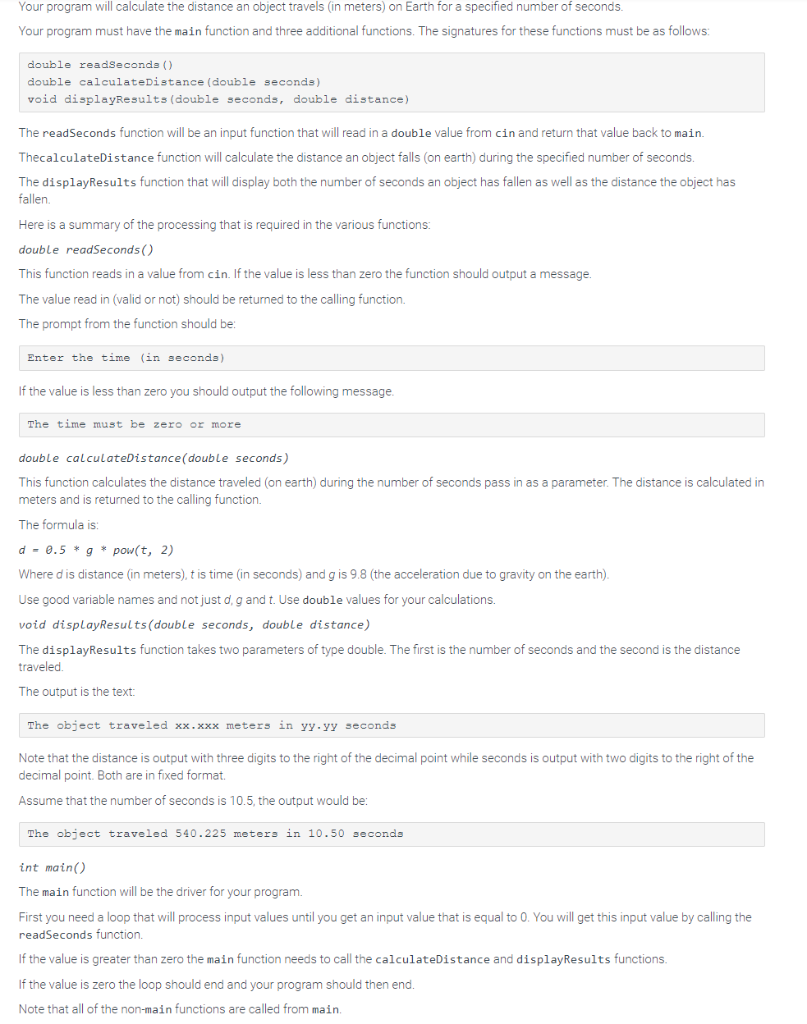In the image, there is a page featuring a list of words. On the left-hand side of the page, there is a small square labeled "Flag as inappropriate". Below this label, several lines of text outline specifications for a programming task.

The first line reads: "Your program will calculate the distance an object travels in meters on Earth for a specified number of seconds." The subsequent line specifies: "Your program must have the main function and three additional functions." It then lists the required function signatures: `double readSeconds()`, `double calculateDistance(double seconds)`, and `void displayResults(double distance)`.

Further down, a detailed summary explains the processing required in each function. The function `double readSeconds()` is described as reading a value. If the value is less than zero, the function is expected to output a specific message. The summary reiterates: "If the value is less than zero, you should output the following message." 

Finally, the image outlines the `double calculateDistance(double seconds)` function, noting that the distance in meters will be calculated. It specifies that this distance should be output with three decimal digits.